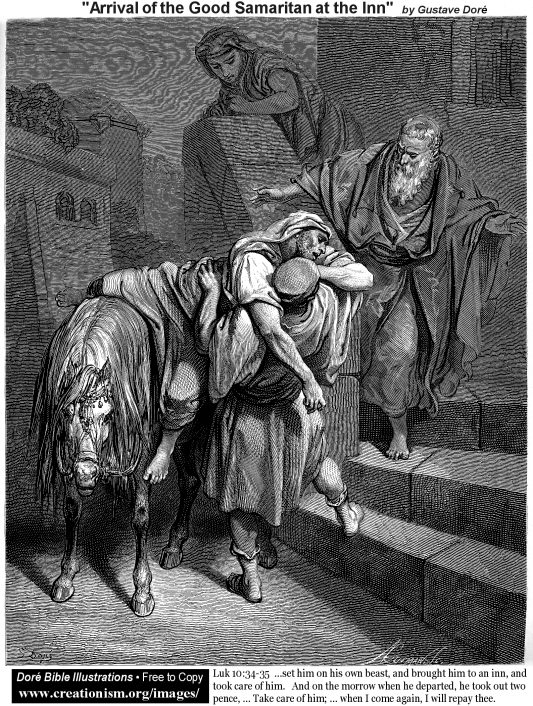The image is a detailed black-and-white woodcut titled "Arrival of the Good Samaritan at the Inn" by Gustave Doré. It shows a scene from the Bible, specifically from Luke 10:34-35, depicted in dramatic monochrome. In the center-left of the artwork, a man is assisting a seemingly exhausted or disabled man off a mule or horse, guiding him toward a series of stone steps. Another bearded man is descending the steps to help, while a third figure stands further back, surveying the scene from a higher position. Surrounding the woodcut, text at the top and bottom of the image provides context and a biblical verse, along with a note that the illustration is free to copy via creationism.org/images. The entire composition captures a moment of compassionate care and aid, rendered in fine detail with various shades of white, gray, and black.